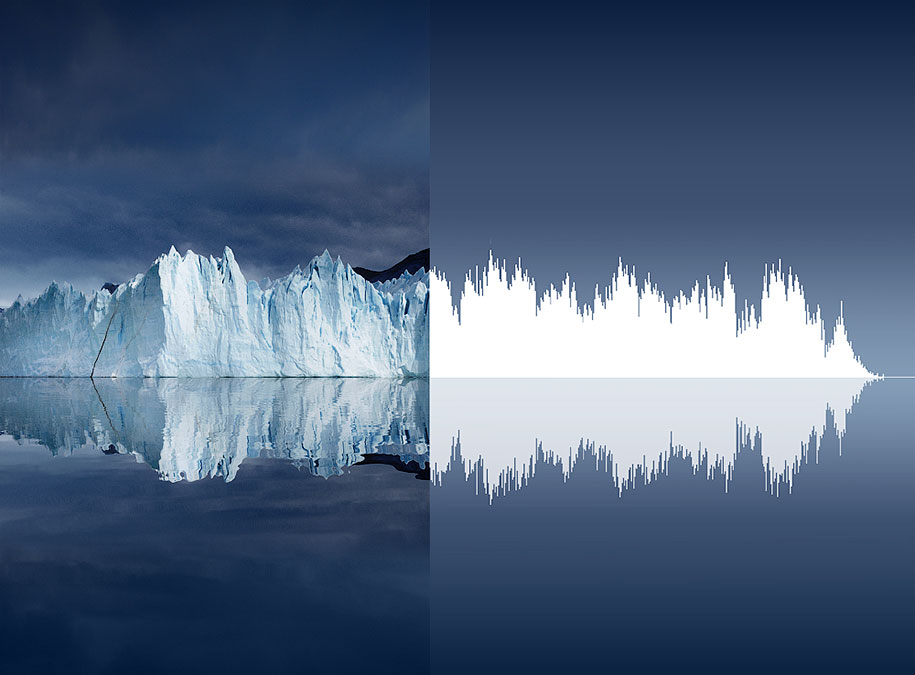This image is a striking piece of artwork divided into two distinct parts. On the left side, it features towering icebergs set against a darkening sky, suggesting the sun has either set or is about to set, casting a dramatic tone. The icebergs display a mix of white and blue-gray shades, and their reflection ripples in the wave-kissed ocean beneath them, adding depth and realism. On the right side, the scene transforms: the icebergs are represented as solid white sound waves or earthquake readings, mimicking the jagged peaks and valleys of the ice formations. Set against a solid bluish background, this side lacks the textured detail of the ocean but mirrors the left side's overall shape and reflection, creating an intriguing blend of nature’s grandeur and abstract representation.